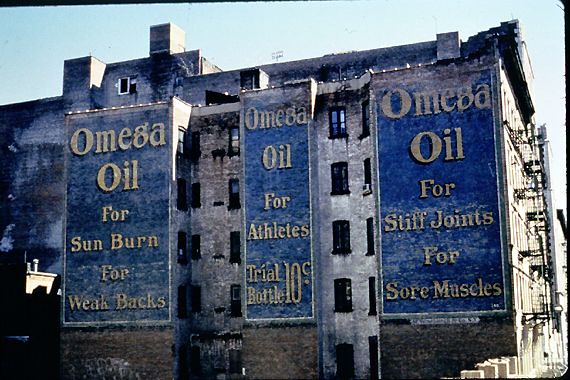The image depicts a very old and run-down building with a faded concrete facade, standing approximately five stories high. The building, appearing dirty with dark areas and windows, features three long, weathered blue advertisement panels running down its side. Each panel is adorned with large, yellow font. The first panel promotes Omega Oil for sunburn and weak backs. The second panel advertises Omega Oil for athletes, mentioning a trial bottle for 10 cents. The third panel highlights Omega Oil for stiff joints and sore muscles. The light blue sky in the background is clear, adding a touch of contrast to the somber, industrial demeanor of the building and its vintage advertisements.